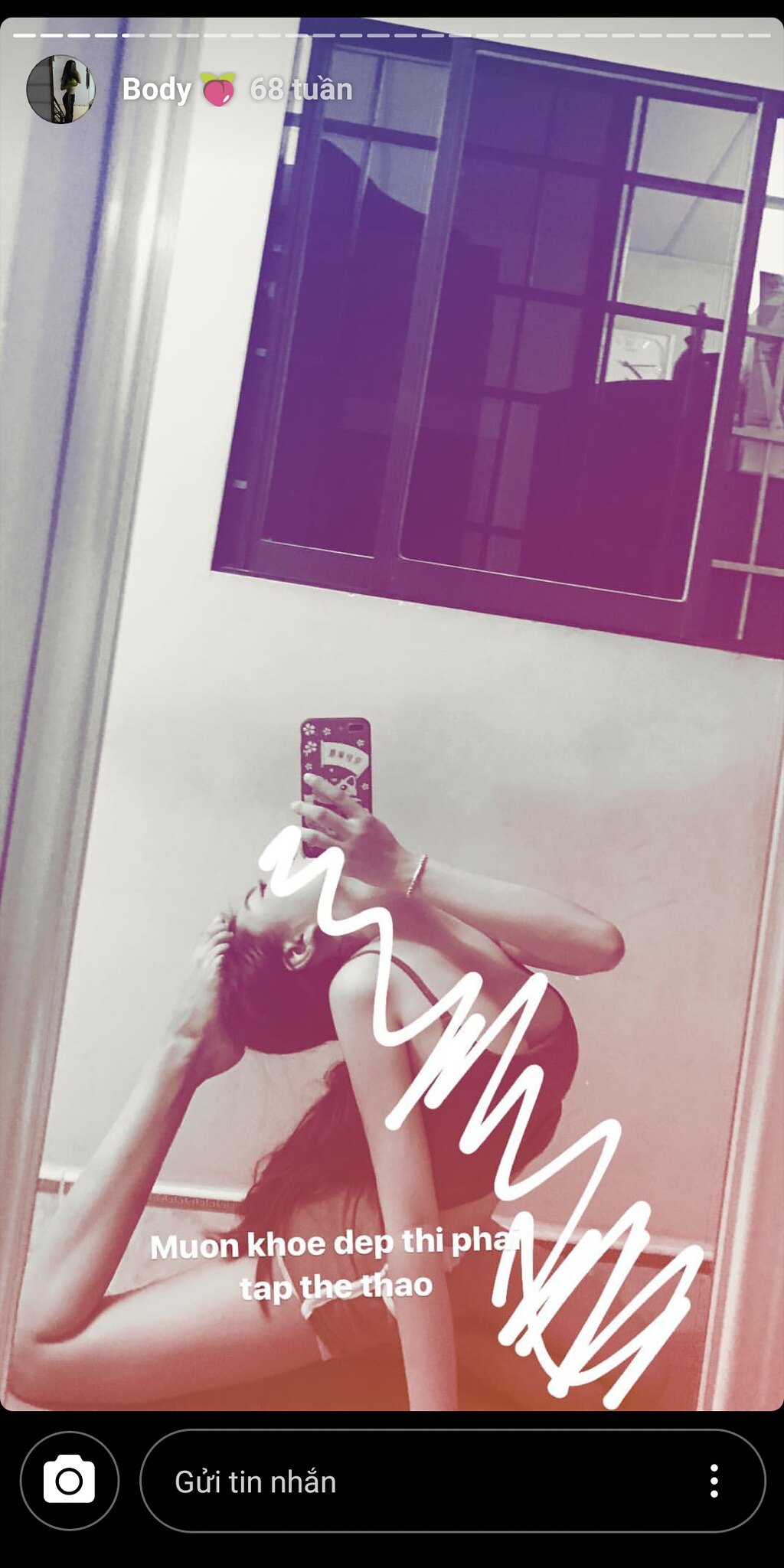The image is a detailed social media screenshot showcasing an acrobatic woman in a small, white room. She is positioned in front of a paneled mirror, executing a contortion where she is bent backward, with her leg lifted over her head and her foot resting on the back of her skull. This creates an arch with her body as she supports herself with one arm stretched on the ground, while the other arm is bent to hold a phone for a selfie. She is dressed in short shorts and a black spaghetti strap tank top, with long black hair cascading down. Notably, there are white scribbles accentuating parts of her face, chest, and leg. The top left corner of the screenshot includes the text "body" followed by colorful lines suggesting stories with hues transitioning from orange at the bottom through black and white to pink and purplish blue at the top, with darker colors towards the peak. There is also an Asian language text overlay comprising of "M-U-O-N K-H-O-E D-E-P T-H-I P-H-A" and "T-A-P T-H-E T-H-A-O". The bottom of the image features a black bar with an icon for taking pictures and space for comments, highlighting typical features of social media interfacing.